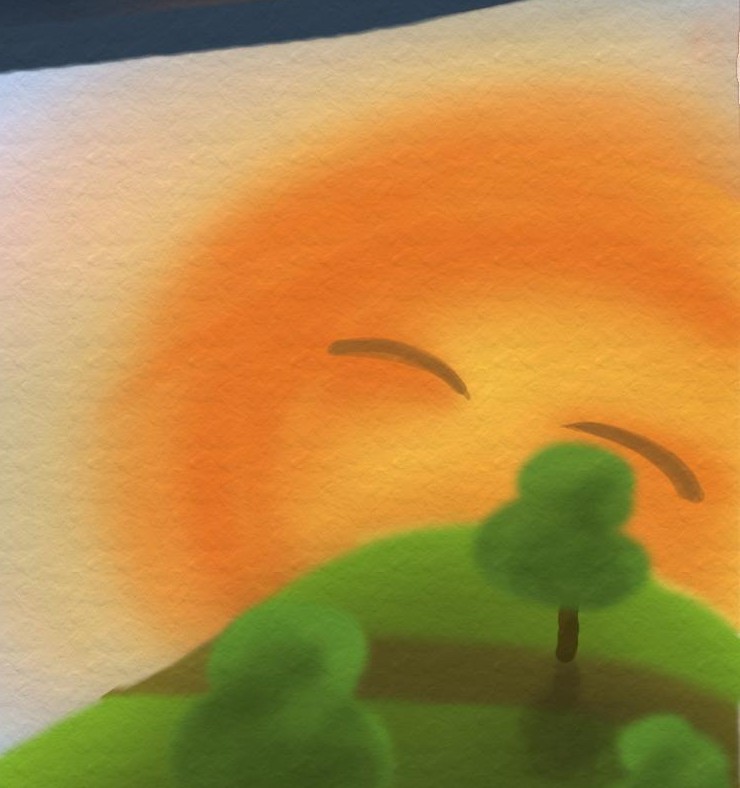This is a close-up, angled photograph of an artistic illustration, painted on a highly textured, porous paper or parchment. Dominating the scene is a large, radiant sun characterized by a circular shape with blended hues of orange and yellow, and subtle, closed eyes that evoke a serene, joyous expression. The sun, devoid of rays, gently floats above a verdant hill, casting a soft shadow over the landscape. The lush green hill, situated on the right side of the image, is traversed by a narrow brown path and adorned with simple yet charming trees. The trees have rounded, green tops and dark brown trunks, with one complete tree prominently visible and the others partially shown at the bottom. The textured paper adds richness to the image, enhancing the visual delight of this whimsical scene.